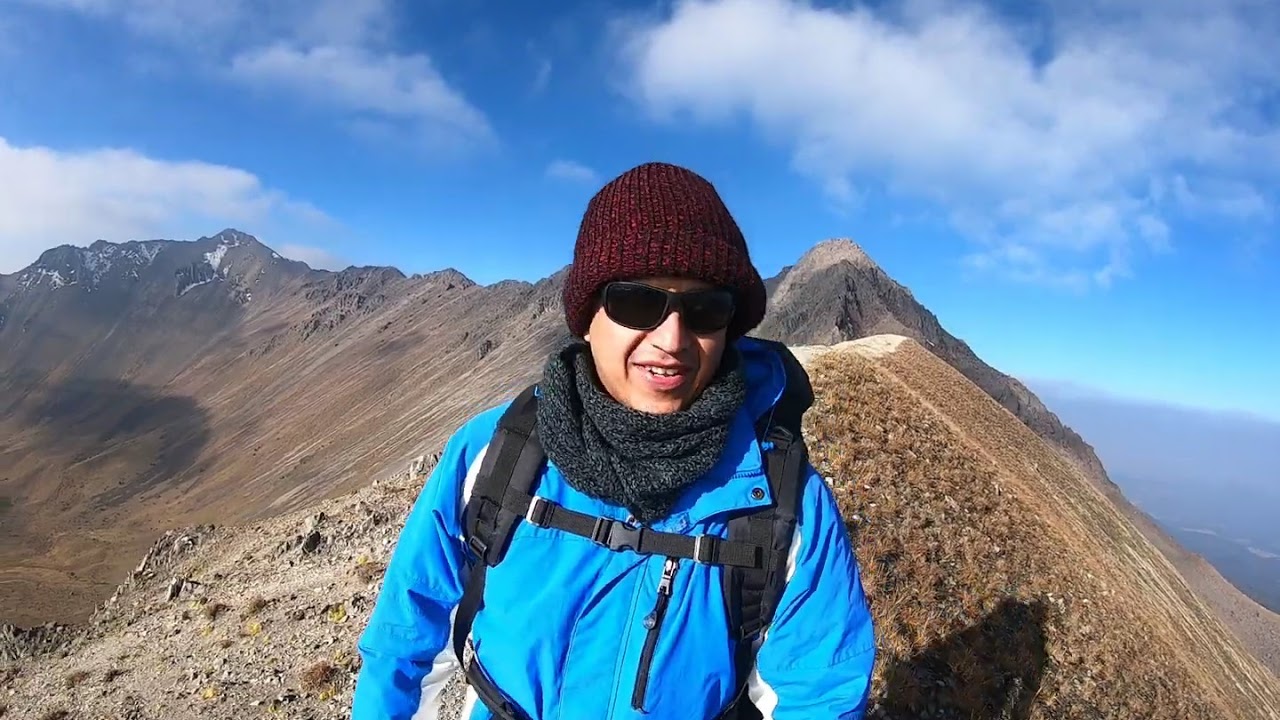The image captures a selfie of a woman standing triumphantly at the top of a high mountain. She's dressed warmly for the adventure, donning a light blue and white jacket, a gray knitted scarf around her neck, a red knitted cap, and black sunglasses with dark lenses. A black backpack is strapped securely across her chest. She appears to be enjoying the moment, perhaps squinting slightly due to the bright, angled sunlight that suggests an early morning climb.

The sky above is a stunning gradient of dark and light blue, punctuated by a few fluffy white clouds. Below her and stretching into the distance, the rugged mountainous terrain unfolds, featuring a nearly vegetation-free landscape dominated by steep, rocky ridges. Shadow patterns from the passing clouds dance across the ridges, adding depth and contrast to the scene. In the far distance, the mountain caps are dusted with snow, signifying the high elevation. To the bottom right, a river snakes through a deep valley, its presence highlighting the sheer magnificence and scale of the landscape. The overall scene conveys a sense of solitude, vastness, and the rugged beauty of nature.